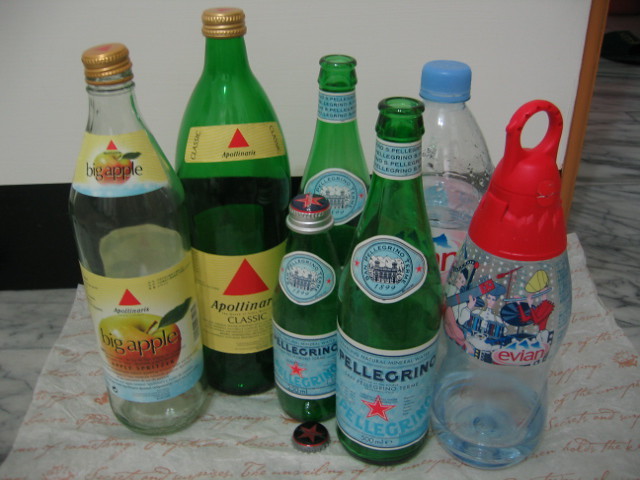This close-up photograph showcases a collection of seven bottles arranged on a sheet of tissue or parchment paper with visible yet indistinct lettering. The background features a white wall accented with light brown wood and a black grating at the bottom. The marble countertop beneath the bottles is white with black streaks.

On the far left, there is a glass bottle labeled "Big Apple," adorned with apple imagery and a distinctive yellow-to-reddish-orange gradient design. Right next to it is a green bottle labeled "Classic" with a yellow and blue label, also featuring a red triangle.

The center of the image displays three green Pellegrino bottles: two tall ones and one smaller single-serve bottle. The smaller bottle retains its silver cap adorned with a red star.

On the right side, two Evian water bottles are present. One has a distinctive red cap with a loop, showcasing design elements like mountains and figures, while the other is a standard clear plastic bottle with a blue cap.

This detailed scene captures a variety of both glass and plastic bottles, emphasizing their unique labels and designs against a subtly textured marble countertop backdrop.